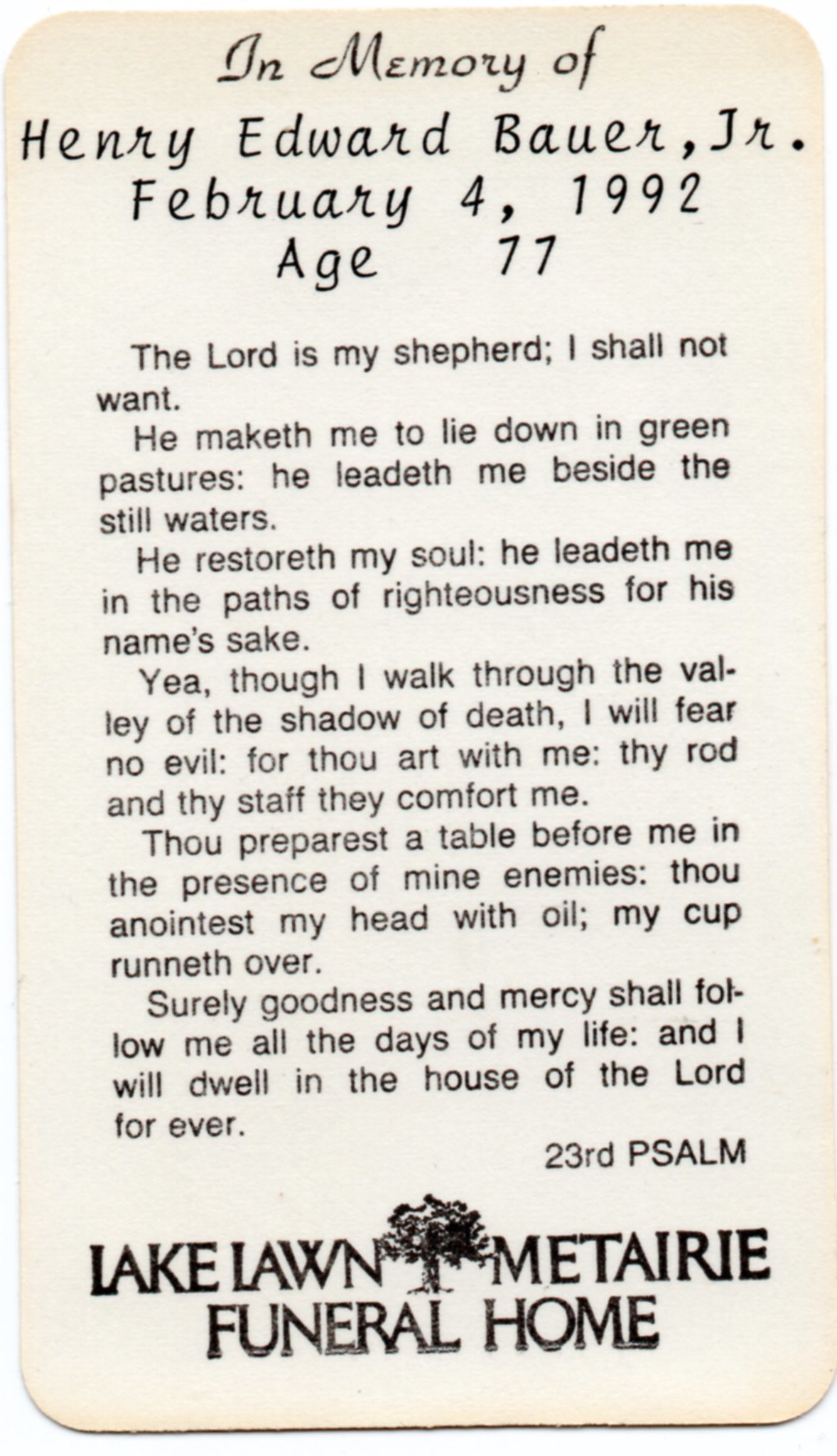This portrait-sized, rectangular memorial card with rounded corners features a creamy white background and black text, framed by a subtle grayish hue. At the top, in elegant black cursive, it reads, "In memory of Henry Edward Bower Jr., February 4th, 1992, age 77." Beneath this heading is the full text of the 23rd Psalm, gracefully printed in a standard black font: "The Lord is my shepherd; I shall not want. He maketh me to lie down in green pastures: he leadeth me beside the still waters. He restoreth my soul: he leadeth me in the paths of righteousness for his name's sake. Yea, though I walk through the valley of the shadow of death, I will fear no evil: for thou art with me; thy rod and thy staff they comfort me. Thou preparest a table before me in the presence of mine enemies: thou anointest my head with oil; my cup runneth over. Surely goodness and mercy shall follow me all the days of my life: and I will dwell in the house of the Lord forever." The bottom right corner bears the words "23rd Psalm." Finally, at the very bottom, the emblem of a tree accompanied by the text "Lake Lawn" and "Funeral Home" indicates the establishment responsible for this solemn tribute.